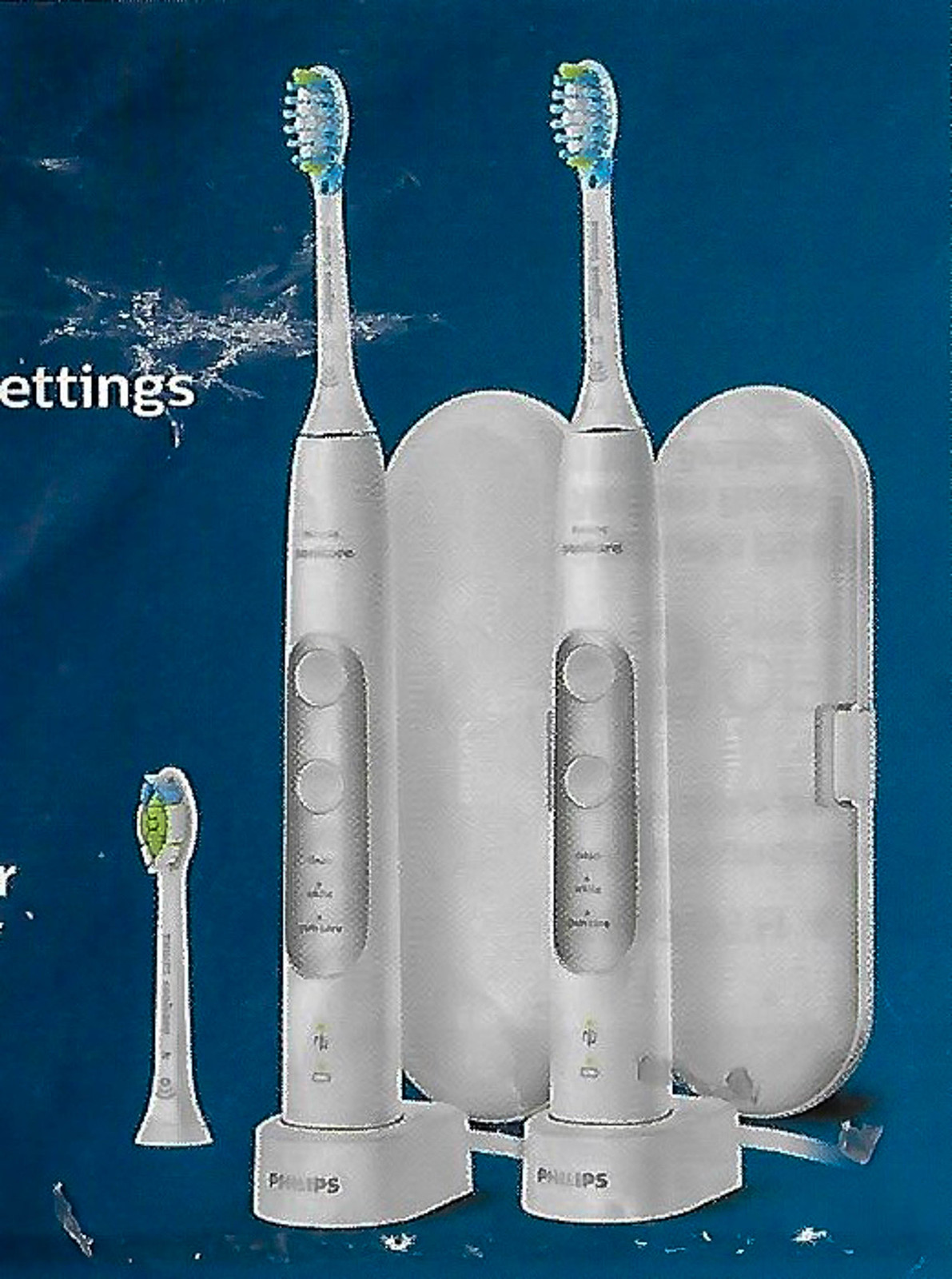The image appears to be an advertisement from a brochure or poster for Philips rechargeable electric toothbrushes, featuring a detailed drawing rather than a photograph. Set against a dark blue background with scattered white streaks and specks, the ad showcases two white Philips Sonicare toothbrushes standing upright on a shared white base that reads "Philips" in gray lettering. Above and partially cut off, the word "Ettings" is visible in white font across the center, possibly a part of the word "settings."

The toothbrushes feature handles with silver oval-shaped areas indicating control settings. Both toothbrushes have brush heads with a color scheme of blue, green, and white bristles. An extra brush head is placed to the lower left corner of the base, matching the attached heads. Behind each toothbrush stands a white oval-shaped clamshell case with a clasp, designed for travel. The overall design hints at elegance and practical utility, reinforced by the attention to detail in the depiction of the product and its accessories.